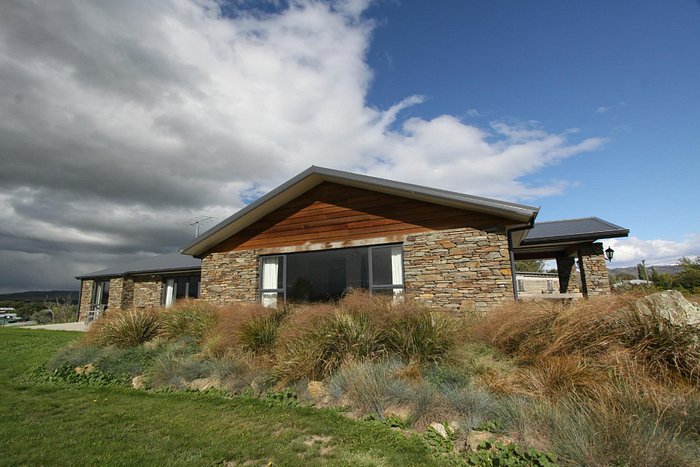The image depicts a picturesque country home, likely situated in a western landscape like Colorado or Wyoming, possibly inferred from the surrounding low-lying hills and mountains. The house is a charming combination of stone and wood, featuring large bay windows that invite natural light. The roof is a mix of peaked and flat sections, finished in brown. An overhang porch, resembling a carport, is visible on the right-hand side, with a car parked in the distance. The foreground boasts a well-manicured, mowed lawn punctuated by wild grasses and small rocks. The sky above is a dramatic gradient, with clear blue on the right transitioning to puffy white cumulus clouds in the center, which darken to stormy gray as they move left. The overall scene captures a serene but dynamic atmosphere, with an emphasis on the expansive sky and the rustic beauty of the house and its surroundings.